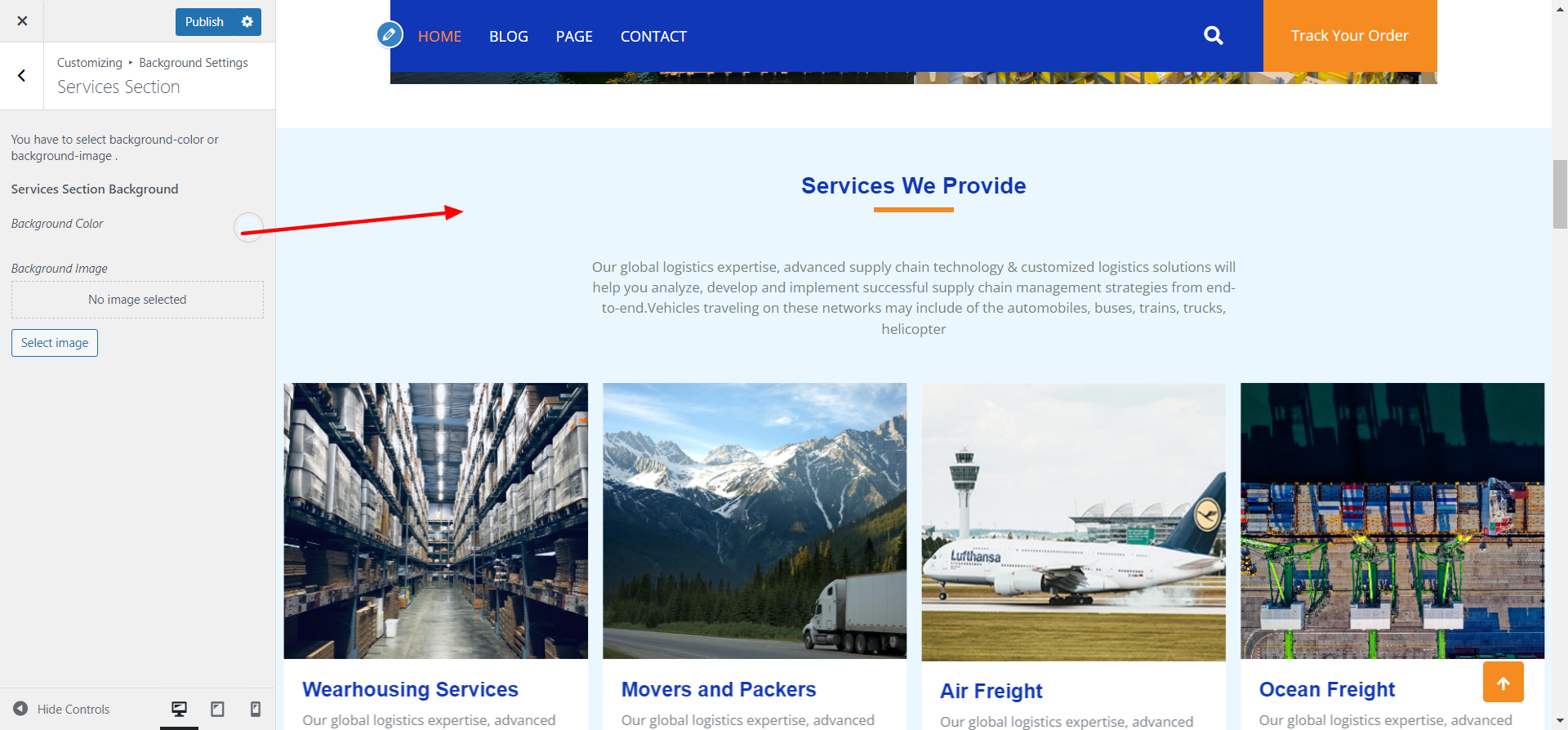A comprehensive view of a computer screen featuring a user interface. At the top left, there is a small bar labeled "Publish" which can be clicked. Below, a section titled "Service Selection" presents various choices, one of which is highlighted with an arrow pointing to it and labeled "Services We Provide."

Dominating approximately 70% of the top, a blue banner spans the screen, transitioning to an orange tab on the right. The blue portion resembles the shade associated with the University of Florida. On the blue section, there is an orange-colored "Home" button, likely the current selection. Adjacent to it, in white text, are options for "Blog," "Page," "Contract," and "Contact." The top right corner of the screen features a "Track Your Order" link and a search bar.

Beneath this header, the highlighted "Services We Provide" option reveals a brief description. At the bottom of the screen, four illustrative images showcase the available services: 

1. "Warehousing Services" – Depicted with an image of a massive warehouse.
2. "Movers and Packers" – Represented by a truck driving through mountainous terrain.
3. "Air Freight" – Illustrated with a Lufthansa cargo plane.
4. "Ocean Freight" – Shown with a cargo ship being loaded.